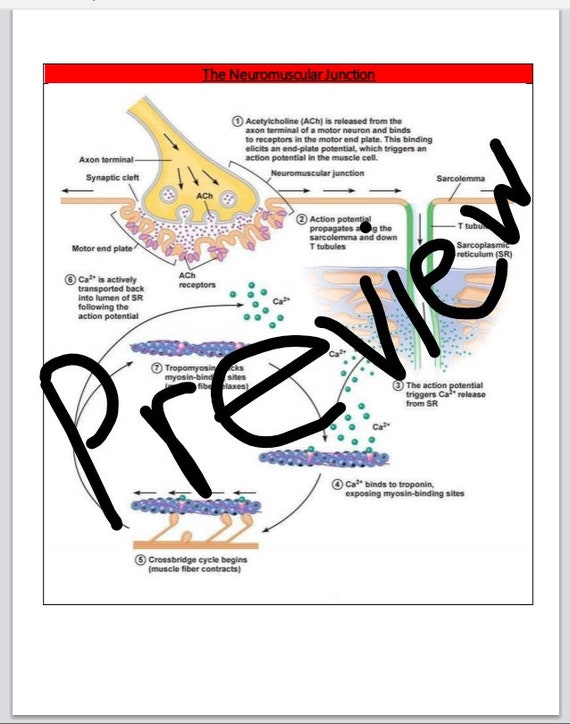This image features an intricately detailed study guide outlined on white paper, with a prominent smaller black square in the center. Topped by a red banner labeled "Neuromuscular Junction," the study guide contains a mix of text, diagrams, and illustrations that explain various components and processes of the neuromuscular junction. Handwritten in black permanent marker across the guide is the word "Preview."

Key elements within the graphic include labeled sections such as the axon terminal, synaptic cleft, ACH receptors, motor end plate, and sarcolemma. The guide illustrates the process where acetylcholine (ACH) is released from the axon terminal of a motor neuron and binds to receptors on the motor endplate. This binding elicits an endplate potential, triggering an action potential in the muscle cell, which in turn causes the release of calcium from the sarcoplasmic reticulum (SR). Calcium then binds with troponin, exposing myosin binding sites necessary for muscle contraction. Numbered bullet points are used to outline each step in the neuromuscular process, although the text is small and detailed, making it difficult to read without close inspection.

Accompanying the text, the visual components include diagrams of neurons and muscle cells, facilitating a comprehensive understanding of the neuromuscular junction's mechanisms. The detailed labeling and clear depiction of the biological processes make this an informative and educational graphic for studying the neuromuscular junction.